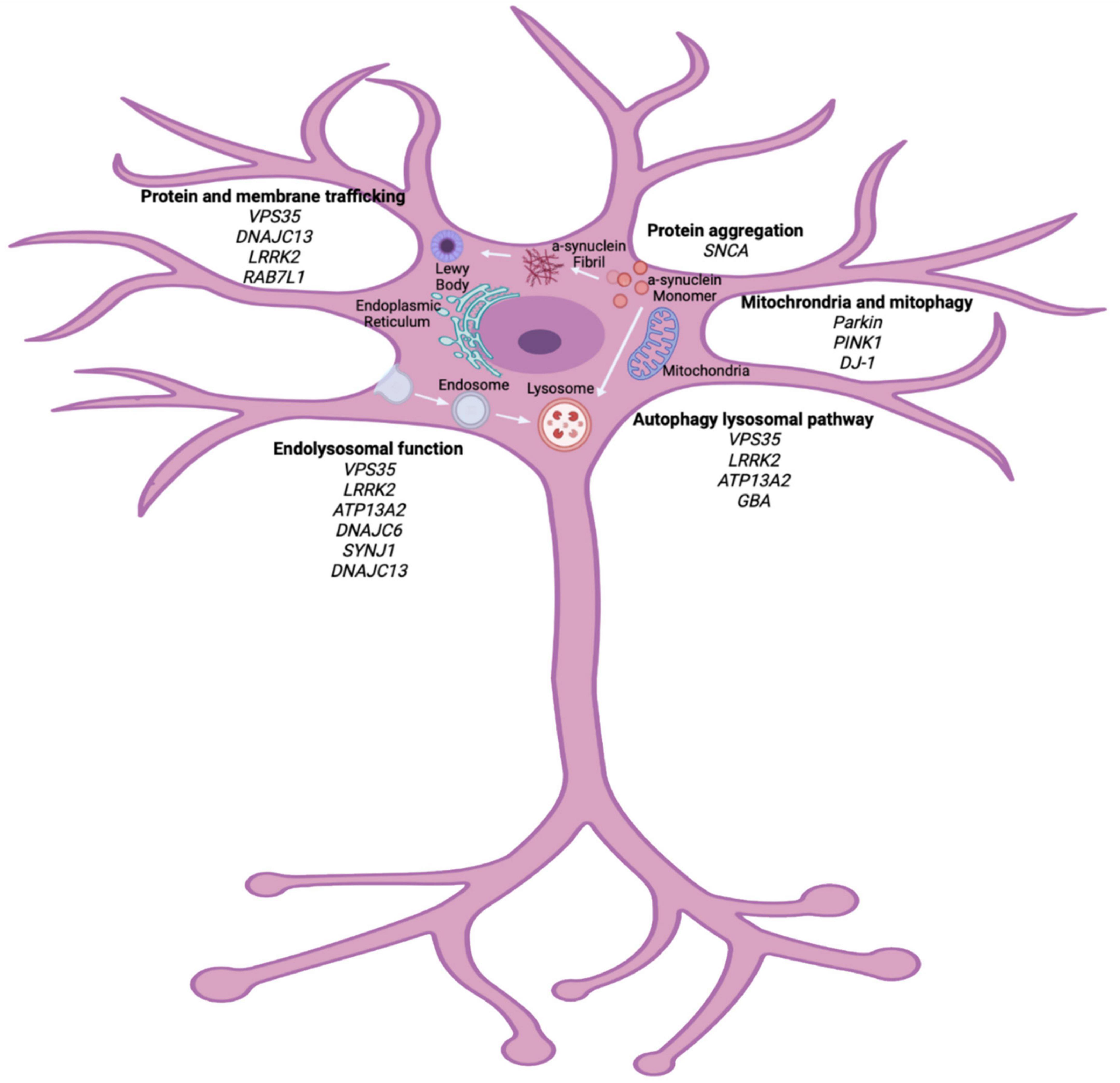The image is an intricate scientific diagram floating on a white background, resembling the shape of a tree with root-like structures at the bottom and branching segments at the top, all shaded in varying shades of purple. The central part of the diagram contains several smaller images, including a round purple shape with a darker purple center, as well as a round figure with an orange outline, a white center, and red and orange dots.

The diagram includes numerous technical terms and labels: 

- **Bottom:** Root-like structures that are part of the diagram.
- **Central Part:** Contains labels such as "endosome," "lysosome," "α-synuclein," "fibro Lewy body," and "endoplasmic reticulum."
- **Upper Left Branch:** Labeled "protein and membrane trafficking" with a series of letters and numbers beneath.
- **Lower Left Branch:** States "endolysosomal function" followed by more alphanumeric codes.
- **Upper Right Branch:** Marked "protein aggregation" with "SNCA" beneath it.
- **Right Middle Branch:** Indicates "mitochondria and mitophagy" followed by "Parkin," "PINK1," and "DJ-1."
- **Lower Right Branch:** Reads "autophagy lysosomal pathway," accompanied by additional numbers and symbols.

The text is written in black and distributed throughout the diagram, enriching the detail and specificity of this scientific illustration. The entire representation seems to convey complex cellular or molecular processes, likely extracted from a science journal or textbook.